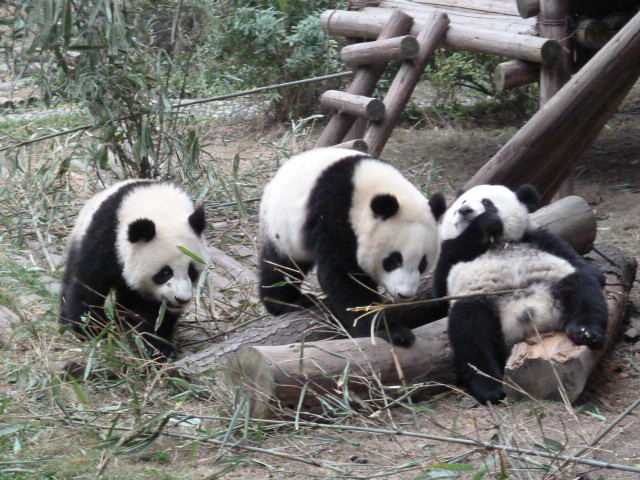This detailed image captures a lively scene with three pandas in their habitat, likely a zoo or sanctuary. The setting is a mix of dirt and patchy grass, interspersed with green and white leaves. Amidst this backdrop are brown, cylindrical logs arranged into a diagonal, ladder-like structure leading to a wooden platform for the pandas to climb.

In the foreground, two pandas are animated: one is traversing grass, heading towards the viewers, while another climbs over a log. The third panda, on the right, offers a stark contrast as it leisurely lounges on its back, head resting on a log and legs propped up on another, exposing its furry, plump belly. The black-and-white coloration typical of pandas is prominently featured, with defining black ears and eye markings standing out against their white faces. Strewn bamboo indicates their diet and adds natural context to the otherwise constructed environment.